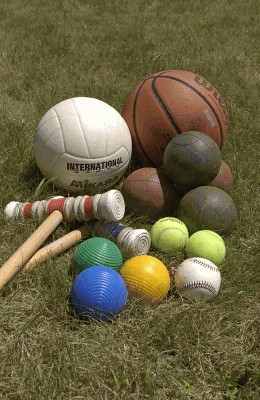The photograph is a detailed, color image showcasing various yard game pieces and sports balls meticulously arranged on a dark green grassy lawn. At the center of the arrangement are three croquet balls in green, blue, and yellow. Just to the right of the croquet balls lies a baseball. Behind the baseball, towards the right, are two yellow tennis balls. Above the tennis balls, two very dark brown, leather-like balls can be seen, resembling coconuts in appearance. Below these are two balls of similar size, colored like a basketball, which also features prominently in the background with its distinct black lines and a visible black Wilson logo. On the left side of the image, a white soccer ball inscribed with the word "international" in black stands out. Between this soccer ball and the croquet balls, two red-and-white croquet mallets with light brown wooden handles are neatly placed. The grass adds a dark, vibrant backdrop to this well-composed and neatly arranged collection of outdoor game equipment, making it ideal as a stock image for promoting activities like a field day or outdoor school events.